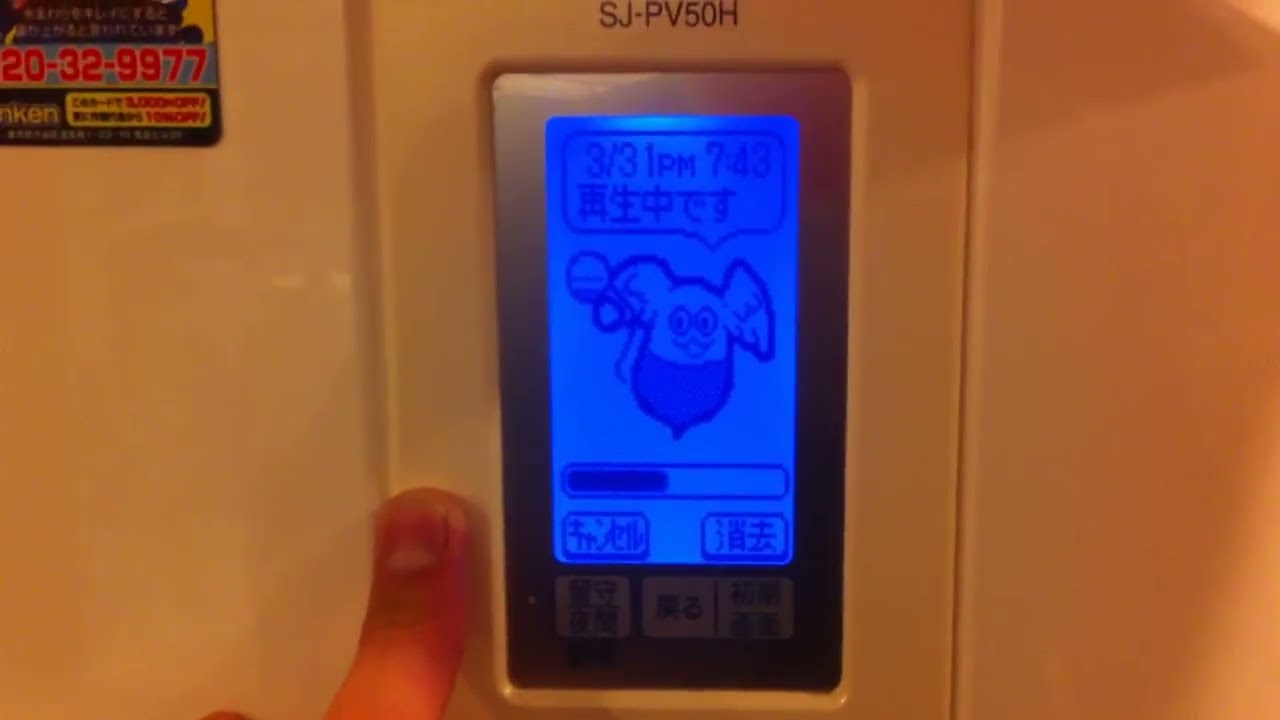A photograph showcases a blue display device with silver metallic borders attached to a cream-colored wall. The device, marked with the model number "SJ-PV50H" in black capital letters on its cream-colored plastic border, features text in a foreign (Asian) language. Prominently, it displays the sequence "3/31 PM 7:43" and a character clip art with a speech bubble. Below this, a blue bar and two additional rectangles containing more foreign text are visible. On the left side of the screen, a person's finger, pressing on the device's border, shows pressure with its tip white and areas below dark red. In the upper left corner, the right edge of a partially visible poster displays the numbers "20-32-9977" in red, followed by additional obscured text.